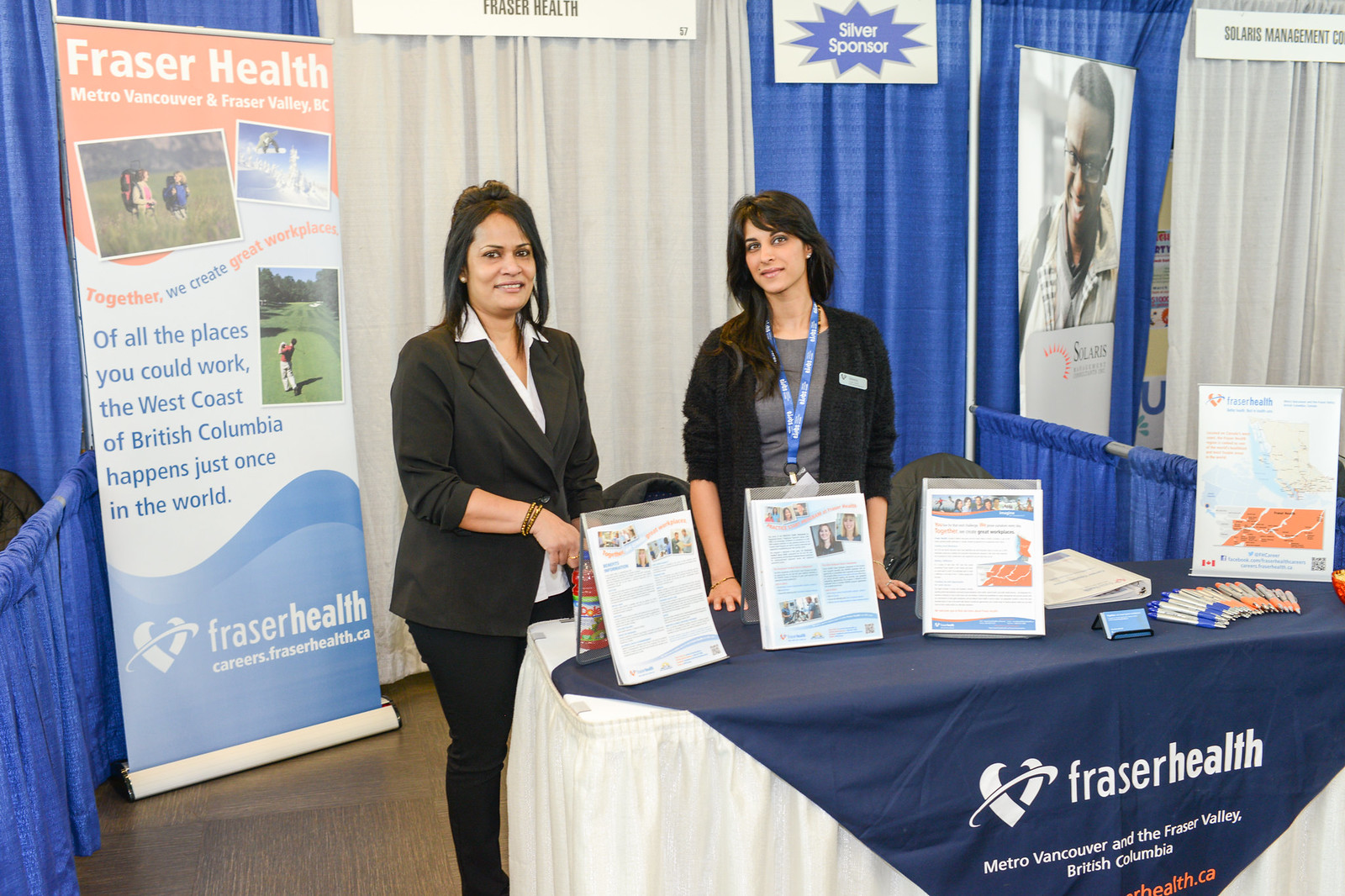The image features a promotional booth for Fraser Health at a conference or event, situated within a setting that includes blue and white elements. Dominating the scene is a table draped with a blue and white tablecloth that prominently displays the Fraser Health logo, along with the regions served: Metro Vancouver and the Fraser Valley of British Columbia. The table is neatly organized with brochures, business cards, binders, and an assortment of pens available for attendees. Standing behind the table are two women, both sporting professional black attire. The woman on the left has shoulder-length black hair and wears a black jacket with black pants, while the woman on the right wears a gray shirt under a black sweater, accentuated by a blue lanyard. Both women are smiling warmly and have conference name cards visible. Behind them, there are multiple banners promoting Fraser Health with an array of activities depicted, such as hiking and golfing. These banners are visually striking, transitioning from orange at the top to white in the middle, and blue at the bottom. The overall ambiance of the booth underscores the organization’s outreach efforts within the West Coast of British Columbia.